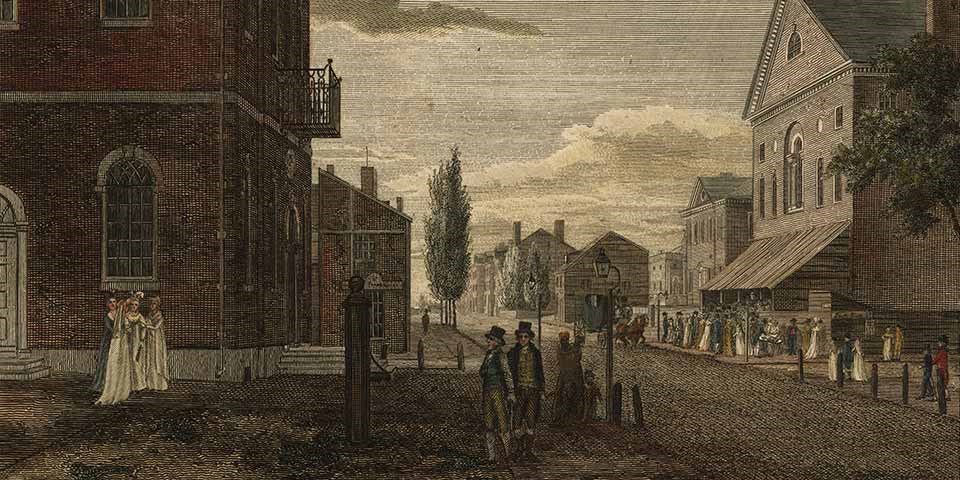This stunning pointillist-style drawing captures an early 20th-century American frontier town, meticulously detailed as though it were a cherished memory brought to life. In the center of the scene, a paved brick road leads the viewer's eye towards the distant horizon, where the sky is filled with a textured expanse of clouds. Tall wooden buildings, some reaching three stories high, line both sides of the street, showcasing the town's well-maintained and somewhat prosperous nature.

To the left, a quaint church stands proudly, adjacent to three women in white dresses, seemingly preparing for a wedding. One of these women might be the bride, perhaps indicated by her prominent position and attire. In striking contrast, another woman wears a long green dress, adding a splash of color to the composition. 

Dominating the middle of the scene are two well-dressed gentlemen, sporting top hats, long-sleeved shirts, pants, and tall boots, epitomizing the fashion of the era. Their prominent positioning suggests they may hold some significance or status in this community. 

On the right side, a large building with an expansive wooden sidewalk teems with life, as a group of about 30 people congregate, dressed in similar period attire. Behind them, a lush tall tree and several others frame the right side of the image, completing the backdrop.

The illustration captures the essence of a vibrant, well-tended frontier town, a nostalgic glimpse into a bygone era, where every detail, down to the horse carriage making its way down the street, speaks of a community rich in both history and life. Though not confined to black and white, the muted, tinted colors add an air of antiquity and charm to the picturesque scene.